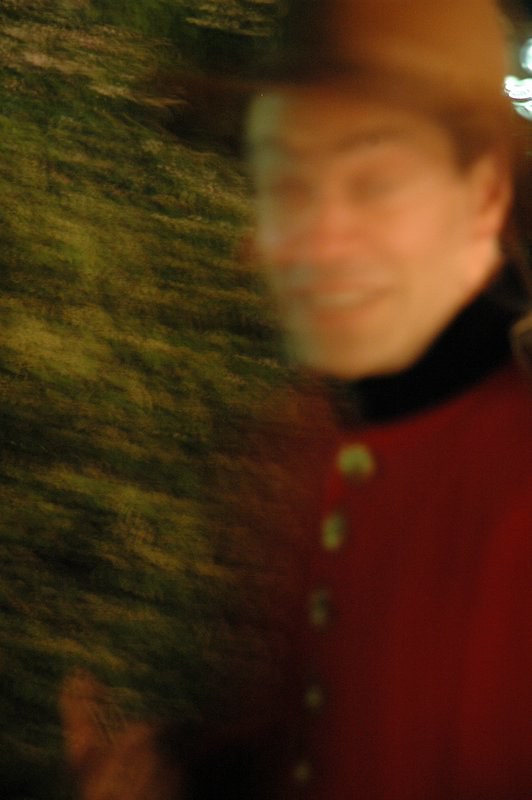In this out-of-focus image, the subject appears to be a Mountie. They are dressed in a distinctive red uniform adorned with yellow buttons running vertically from the collar down the chest. The neck is wrapped in a black fabric, possibly a functional part of their uniform. The Mountie faces the camera in a relaxed demeanor, with their eyelids gently closed and a faint smile revealing their teeth and lips. Their facial hair is stubbly, adding a rugged touch to their appearance. The nose has a pinkish hue, and the right ear is visible while the left side of the background predominantly features green leaves. A brown hat sits atop their head, and the right eyebrow is slightly raised, giving more character to their expression.